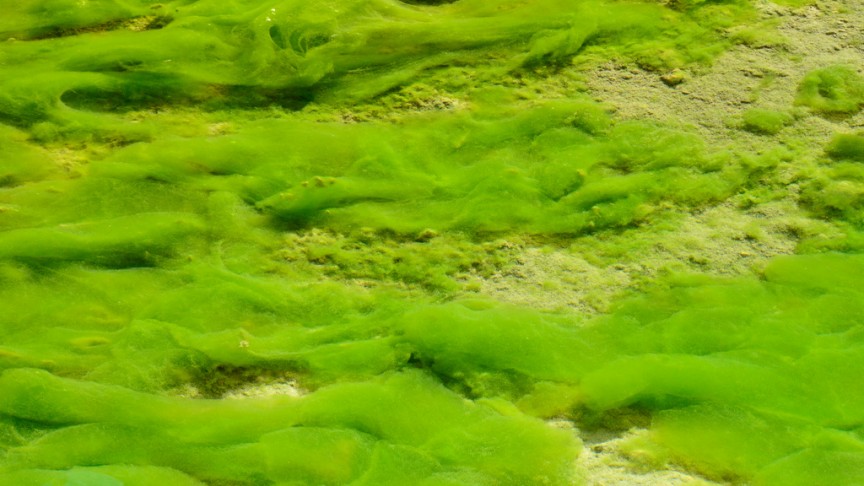The image showcases a bird's eye view of an uneven piece of green land, which appears to be an intricate landscape of algae with varying shades of green. The green land is dotted with regions of wispy, three-dimensional green fuzz, creating a textured and multi-layered appearance. The vibrant, bright green algae predominantly covers the image, with thicker, cloud-like patches concentrated towards the left, middle, and bottom corners. These dense algae formations obscure parts of the underlying surface, which seems to be light-colored sand that peeks through, particularly at the top right and bottom right. The algae transitions from darker green on the left to lighter green on the right, where it becomes less thick, revealing more of the sandy, powdery ground beneath. These lighter patches exhibit a more yellowish-green hue, enhancing the dynamic visual complexity of the scene. The overall effect is a visually striking contrast between the lush, bright green algae and the sparse, dry, and powdery areas.